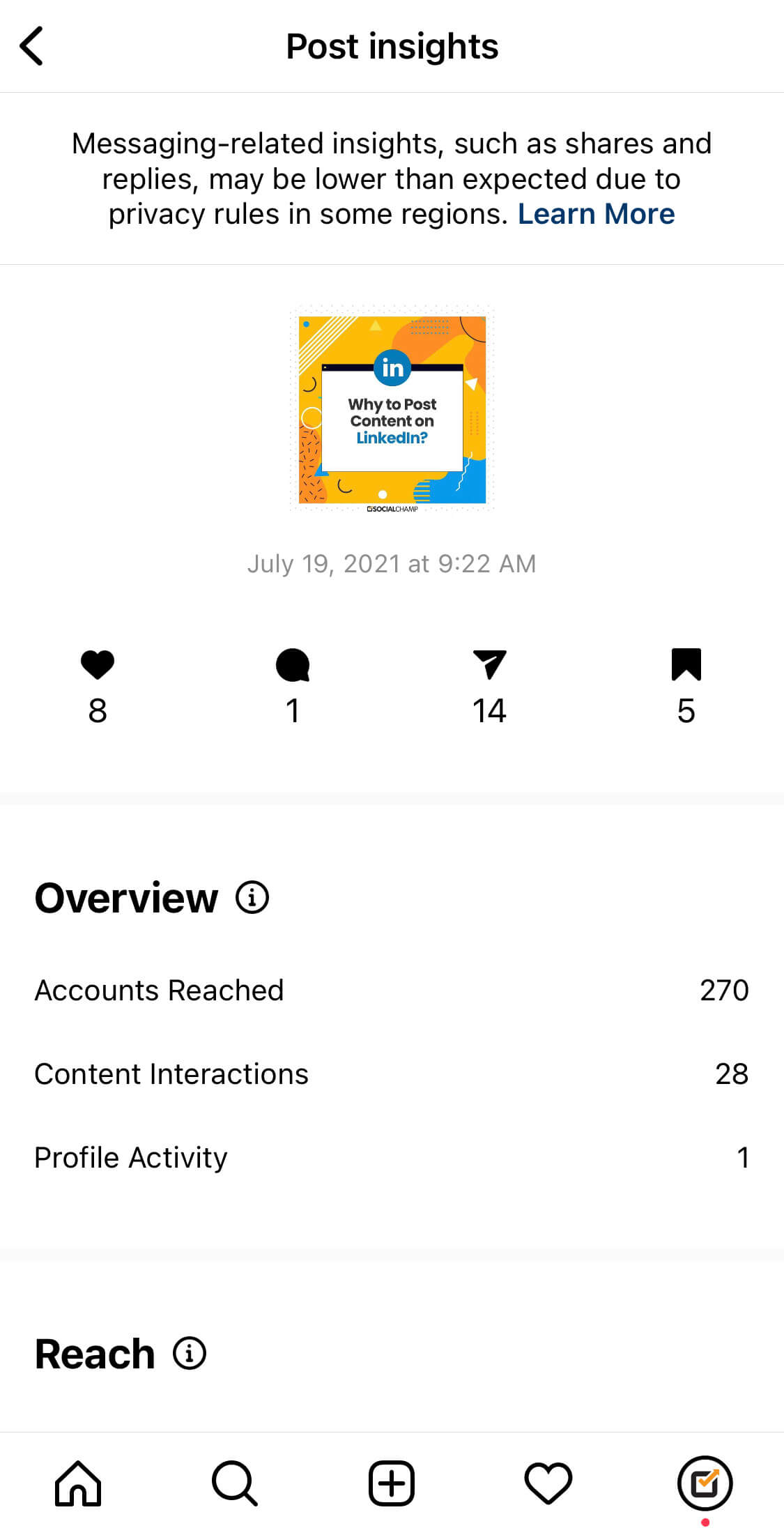Detailed caption:

This image, captured from a mobile device, showcases an analytics page titled "Post Insights." At the top, a notification highlights that messaging-related insights, such as shares and replies, may be lower than expected due to regional privacy regulations. A clickable link labeled "Learn more" in blue allows users to access further information. 

Beneath the notification, an eye-catching graphic features an orangish box with a touch of teal. Within this box, there's a blue circle with the word "in" prominently displayed in white. Below the graphic, a white rectangle with a black-tipped top edge poses the question, "Why to post content on LinkedIn?" with "LinkedIn" highlighted in blue.

The date, July 19th, 2021, along with the time, 9:22 a.m., is displayed further down the page. Engagement metrics show 8 hearts, 1 comment, 14 shares, and 5 banners. An overview section at the bottom provides additional performance data, indicating that the post reached 270 accounts, had 28 content interactions, and generated 1 profile activity.